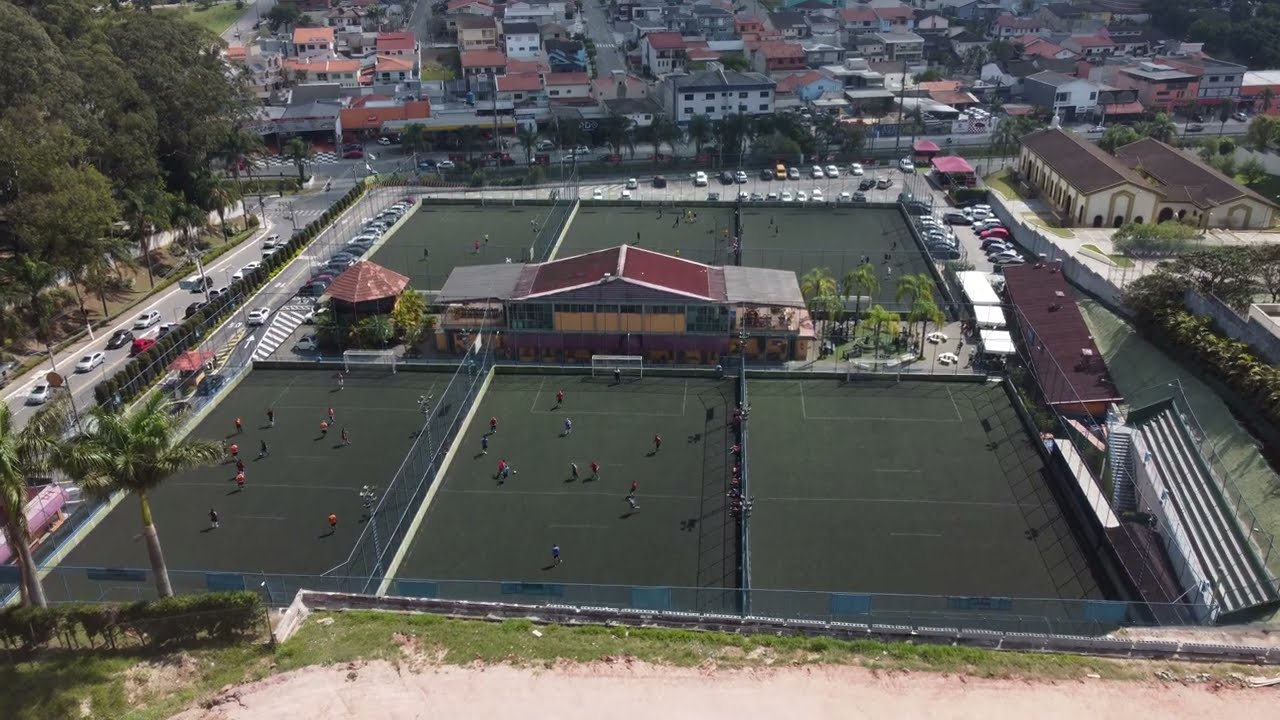The image is a detailed, color aerial photograph in landscape orientation, capturing a bustling urban area centered around a large sports complex with six soccer fields. The fields are organized in two rows of three: the top row has scattered players, while in the bottom row, the left and center fields are active with games while the right field remains empty. A prominent red-roofed building stands at the center of these fields, accompanied by another building to its left with a circular, rusty-red roof. Surrounding the complex, there are parking lots filled with cars, and small spectator stands are visible on either side of the fields. On the right side of the image, there's a residential area with many red-rooftop houses, including a church. A street lines the left side of the complex, bustling with two-way traffic, and is framed by patches of green grass, palm trees, and other foliage. The style of the photograph is representational realism, offering a comprehensive view of the urban sports facility and its surroundings.